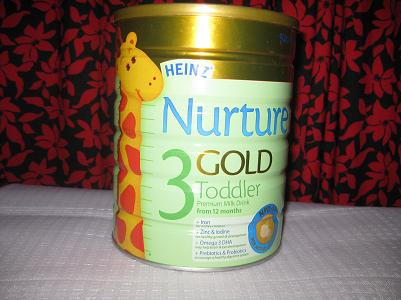The photograph captures a can of Heinz Nurture Gold Toddler 3 formula prominently displayed against a background featuring a black curtain adorned with red flowers. The can, resembling a coffee tin, has an upper gold section including a slightly lighter gold lid, transitioning to a primarily light green label. The brand name "Heinz" and the word "Nurture" are written in blue, with the term "Gold" in gold lettering, and the number "3" as well as the word "Toddler" in green. The label also features a prominent illustration of a yellow giraffe with red spots, its neck spanning down the left side and its head adjacent to the word "Heinz." A small white rectangular diagram on the right side of the can lists additional details, possibly nutritional information like iron and zinc content. The can rests on a white mattress or coverlet, providing a clear, well-lit view of its details.